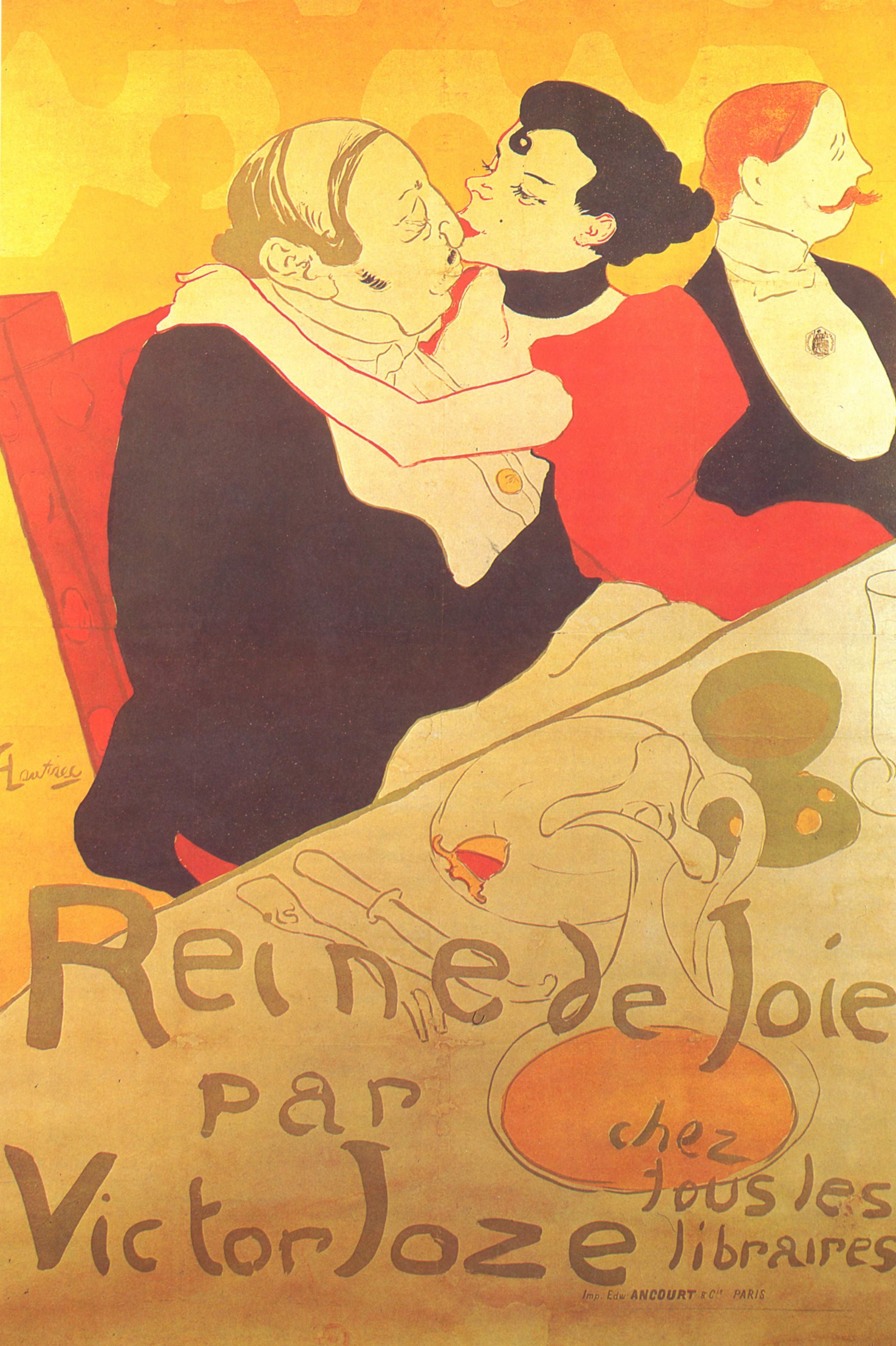This artwork, resembling an Art Deco piece with a restrained color palette of blues, purples, and reds, primarily portrays an intimate dinner scene. In the top half, an older, overweight man with a balding head and closed eyes, dressed in a black penguin-style tuxedo with golden buttons, turns to the right as a woman kisses him on the cheek. The woman, adorned in a red dress and a black scarf, has short black hair styled with a twist forming a circle on her forehead. Her eyes are wide open, and she wears red lipstick accentuating her pointy nose. To their right stands another man with orange hair and a sharp mustache, dressed in a similar tuxedo, also with closed eyes, gazing into the distance. Below these characters lies a dining table set with plates, utensils, a jug with juice, and a knife and fork. Above the table, text reads: "Reine de Joie par Victor José," and in the corner, "Chez Tous Les Libraires."